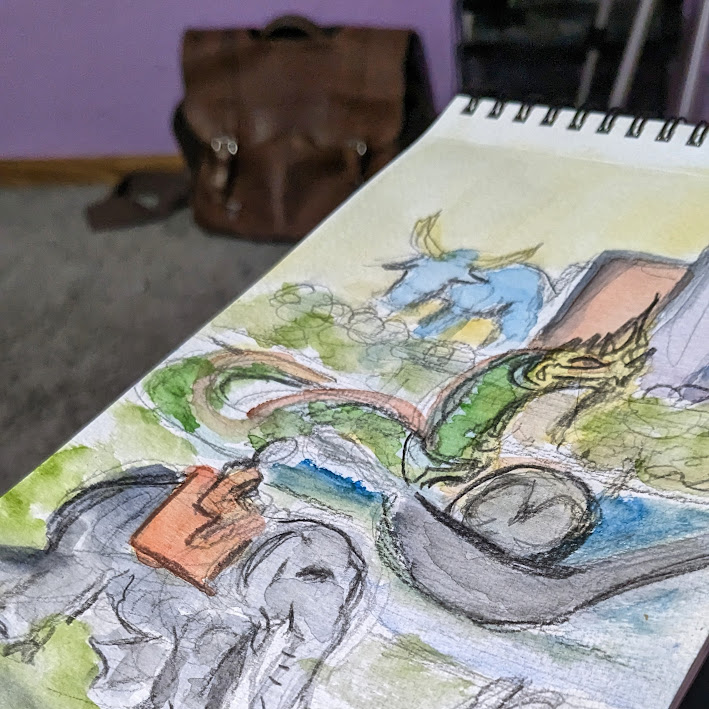The image displays a square-shaped notepad with a black spiral binding at the top. Positioned centrally within the image is a detailed drawing. In the bottom left corner, a gray-colored elephant is depicted with a figure of a person riding on its back. Above the elephant, a long green creature with a yellow head is illustrated, seemingly emerging from water. The drawing combines elements of nature and whimsy, giving the notepad a lively and imaginative appearance.